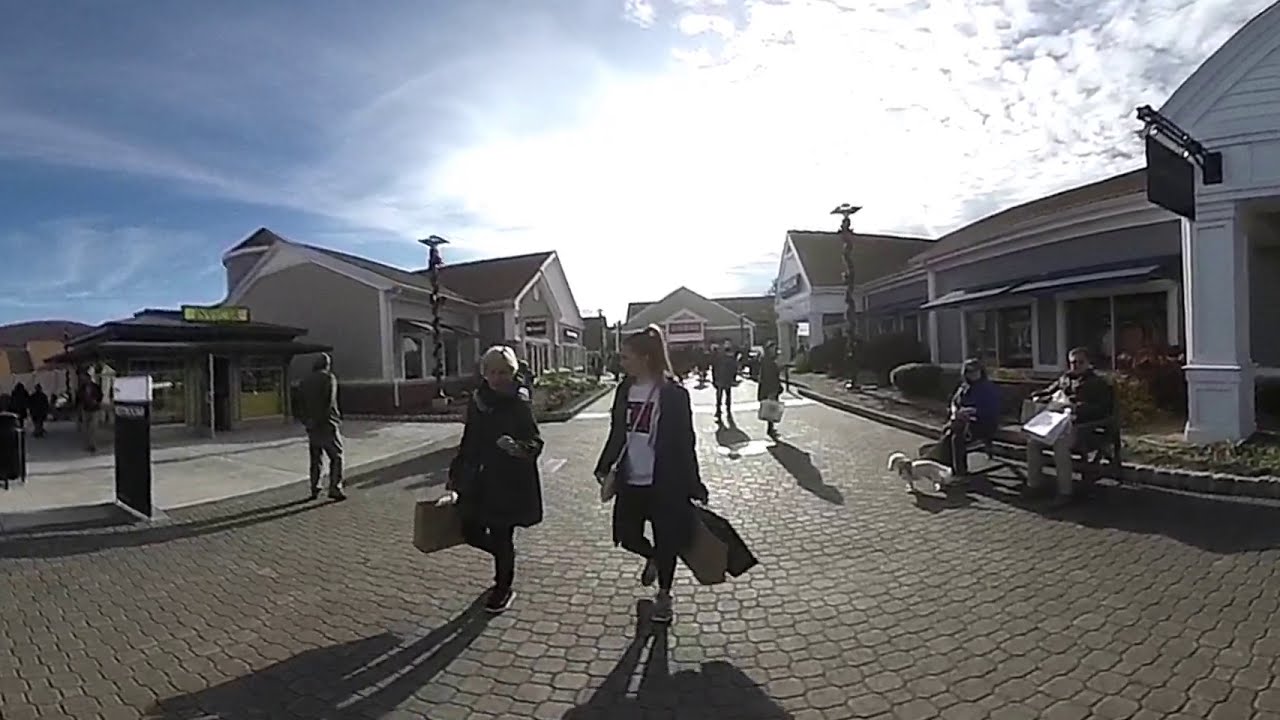This photograph captures a lively scene in an outdoor plaza or shopping center featuring cobblestone tiles beneath the feet of various individuals, amid a backdrop of interconnected storefronts resembling quaint little houses with triangular-shaped roofs. The sky above is a bright blue, accentuated by a few gleaming white clouds with the sun peeking through. Central in the image are two women walking towards the camera, possibly a mother and daughter. The younger woman, appearing to be in her early to mid-20s with a high ponytail, is wearing a white sweatshirt with "USA" printed on it and a raincoat. She carries two paper shopping bags and a purse slung over her shoulder. Beside her, the older woman dons a blue raincoat with a fur collar and also holds a shopping bag, suggesting they have just finished a shopping trip. To the right of the image, two people sit on a bench, one of them holding the leash of a small white dog. Additionally, a solitary man walks on the left side of the photograph. The colors in the scene include an array of black, white, brown, blue, green, yellow, pink, red, along with shades of gray, enhancing the daytime atmosphere.